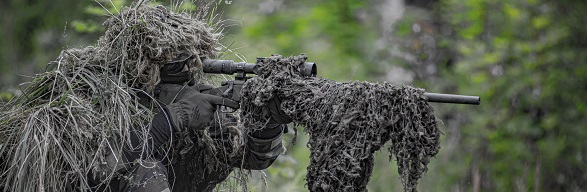The full-color, horizontally rectangular photograph depicts a meticulously staged outdoor scene in natural daylight. The backdrop, a blur of vibrant green foliage, including leaves, branches, and bushes, adds depth and context without drawing focus away from the subject. The primary focus is a well-camouflaged soldier, positioned on the left and facing towards the right, blending seamlessly into the jungle environment. Dressed in an intricate camouflage of dry grass and vegetation, covering his head, shoulders, and back, the soldier wears gray gloves and dark glasses, adding to his concealed appearance. His rifle, equipped with a scope and shrouded in gray netting to prevent glare, points right as he peers through it, seemingly prepared to take a sniper shot. The haunting mood conveys a wartime scenario, where the stealth and precision of the sniper are critical against the lush, green backdrop of the jungle.